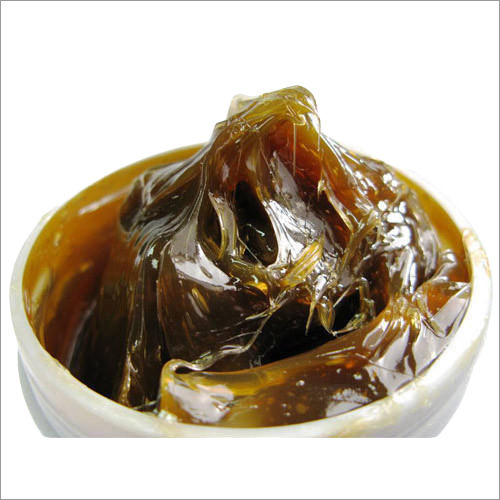The image depicts a circular, off-white plastic container set against a plain white background with a thin black border outlining the entire scene. The container, resembling a small jar or bowl, is filled with a caramel-colored, extremely viscous substance that appears thick and sticky. The material inside varies in shades of rich, dark brown and looks somewhat like hardened melted sugar or caramel, with a texture that has formed into a small peak in the center. Some of this substance seems to be slightly dripping and hardened on the edges, indicating its gooey and sugary nature when heated. The overall appearance suggests it could be a type of confectionery, like caramel, or potentially a product seen in a dispensary, further adding to its enigmatic and multi-purpose visual impression.